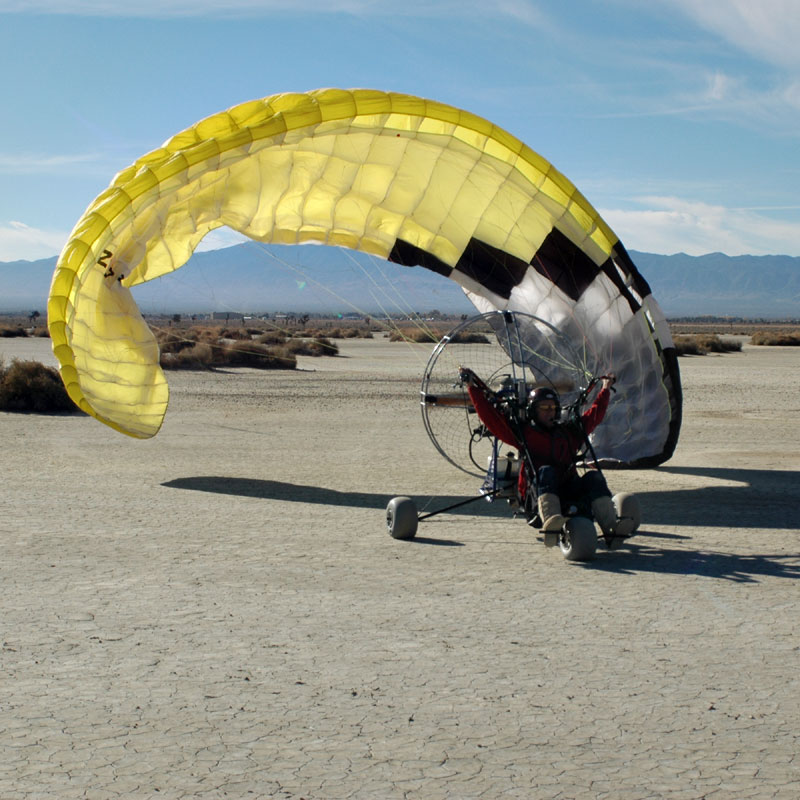This image captures a man in a desert setting, atop a three-wheeled paraglider resembling a go-kart. The vehicle has two rear wheels, a front wheel, and a large fan at the back. The fan appears to propel air into a large parachute, which is adorned with a pattern of yellow and white sections, interspersed with black squares, forming an arch. The man is dressed in a dark jumpsuit with red sleeves, tan boots, and a helmet with sunglasses. He is seated with arms extended, holding onto handles and seemingly directing the parachute. The landscape features a cracked, dusty surface, indicative of a dried lake bed or arid desert environment. Sparse, dying bushes and shrubberies dot the landscape, stretching into an open expanse. In the far distance, tall mountains rise on the horizon, under a clear blue sky. The scene conveys a sense of stillness, as if the paraglider has recently landed or is preparing for takeoff.